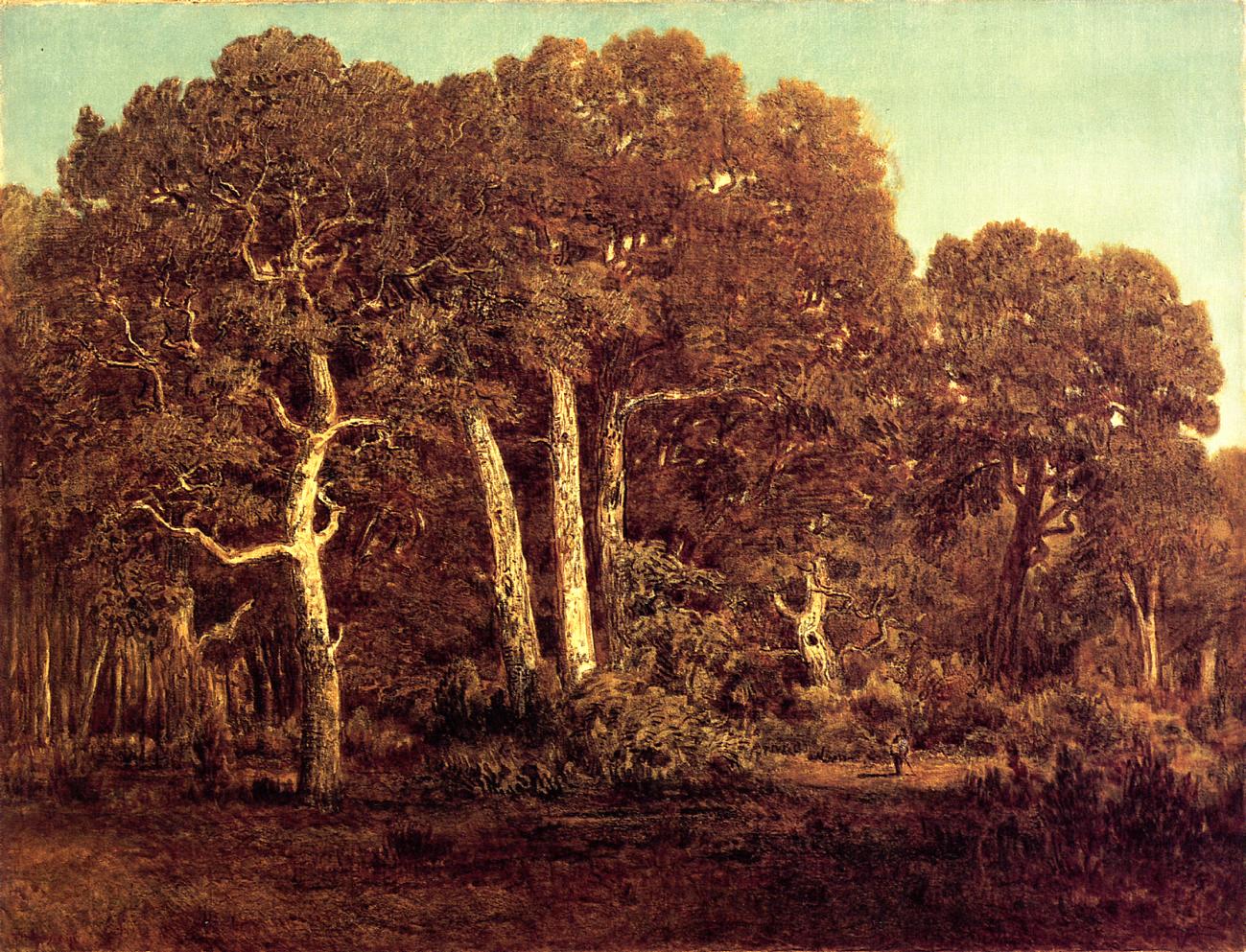In this sepia-toned image, a serene forest scene unfolds, revealing towering oak trees with thick, rust-colored trunks and jagged, sprawling branches that converge into a round, dense canopy. Sunlight filters through the lush greenery, creating dappled light on the grassy land below, which occupies the lower quarter of the image. A small clearing bathed in sunlight appears near the bottom right, where a tiny figure, possibly a man in overalls and a white shirt, stands holding a cane or a walking stick. The clear sky above transitions to a light green hue, adding to the mystical and timeless quality of the painted depiction. The overall impression is that of a tranquil summer or spring day in a dense, thriving forest.